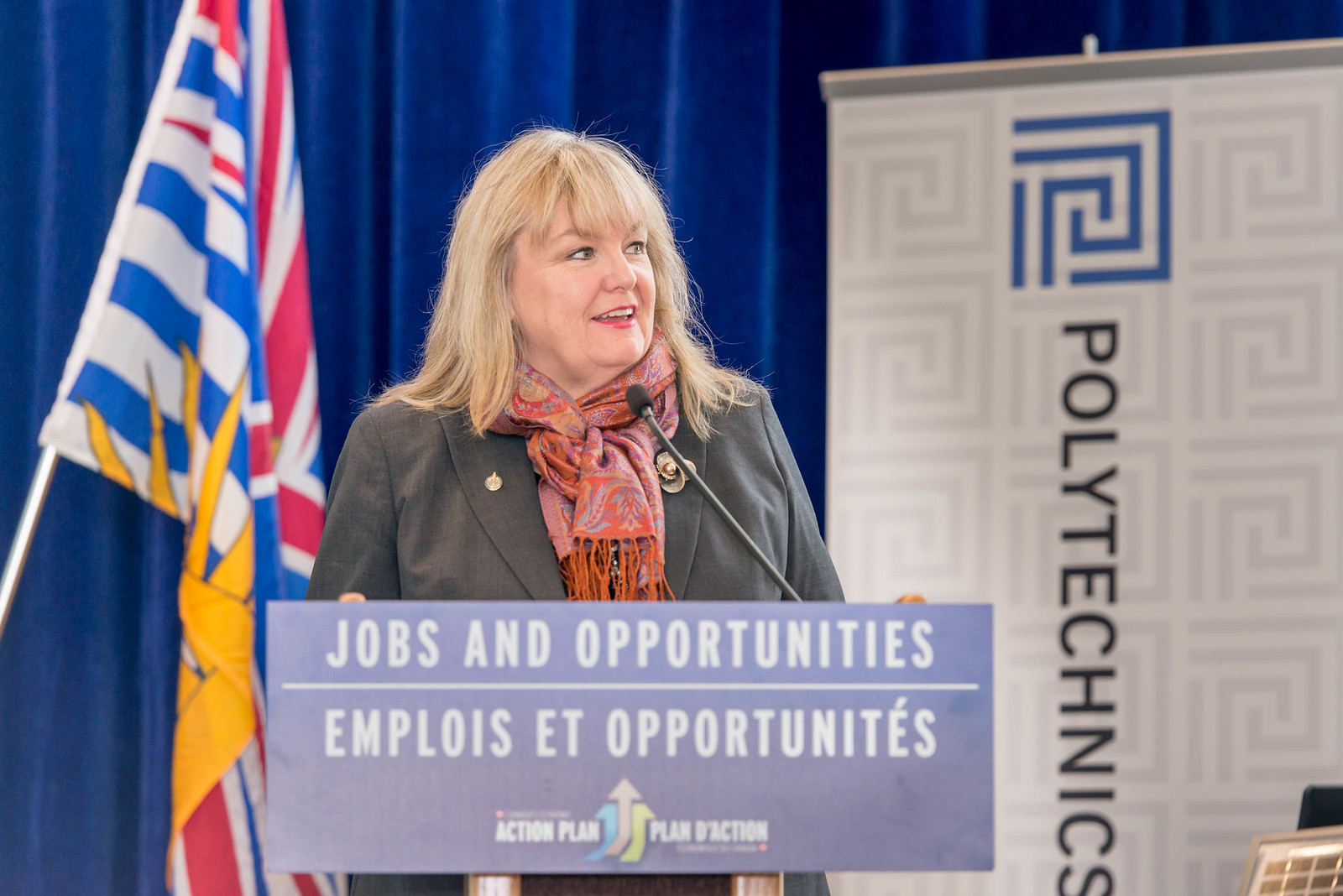This image features a blonde woman speaking at a podium adorned with a sign that reads "Jobs and Opportunities" in English and "Emplois et Opportunités" in French, followed by the phrase "Action Plan - Plan d'action" alongside a logo with three arrows. She is dressed in an olive green suit paired with a paisley scarf around her neck and has a gold pin on her jacket. Behind her is a deep blue curtain, contributing to the formal setting. To the left, there is a colorful flag with red, white, and blue stripes and a yellow sun emblem. On the right, partially cut off, is a white banner with rigid maze-like lines and a blue maze design at the top, featuring the word "Polytechnics" written vertically in bold black text. The composition conveys a professional backdrop, emphasizing themes of employment and education.